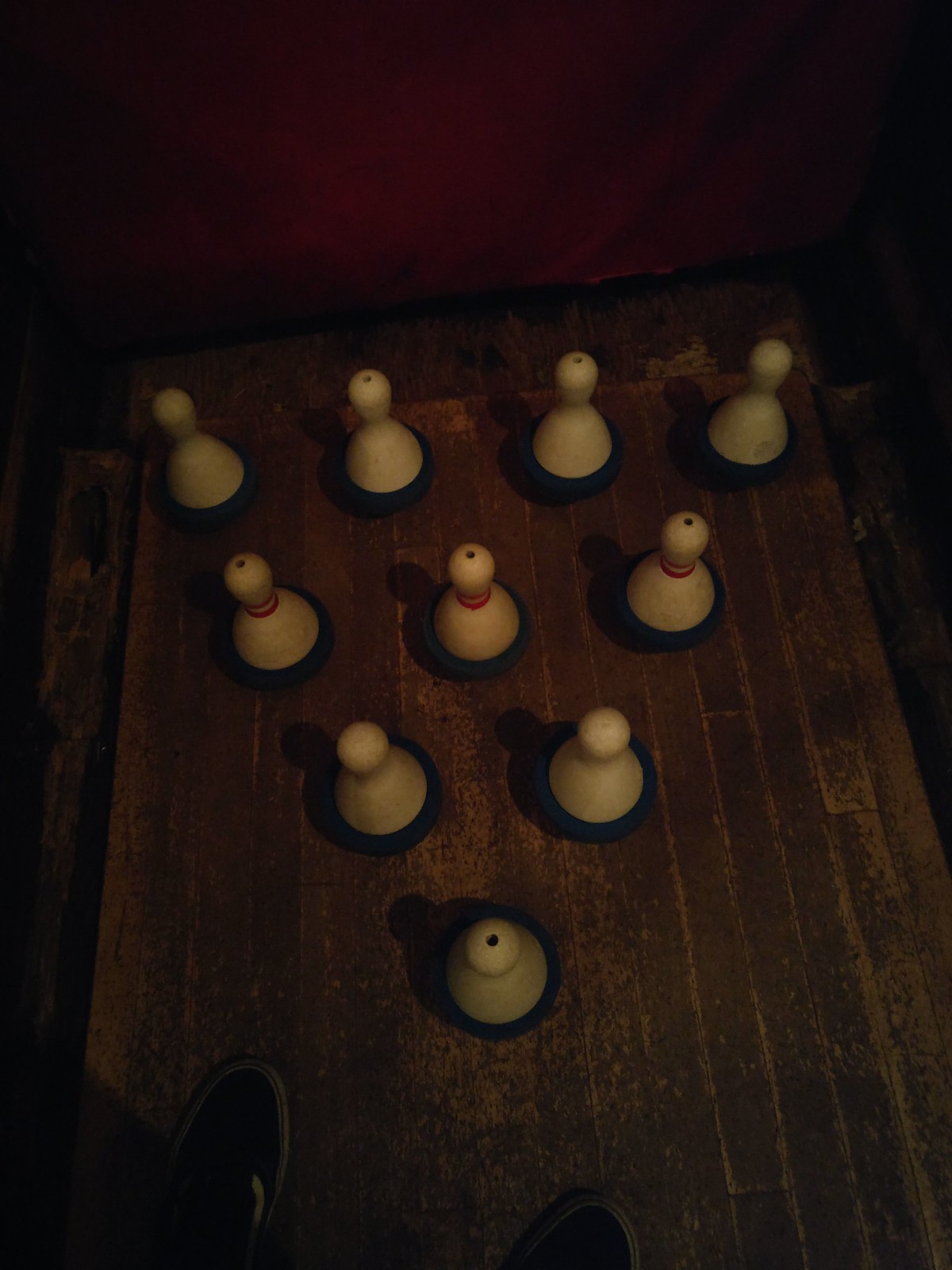This color photograph, taken from above in a dark setting, captures a small game involving ten tiny cylindrical bowling pins on a chocolate brown wooden surface that shows signs of wear. The pins are arranged in an upside-down triangular formation: four in the back row, three in the next, then two, and one at the front. The four pins in the second row feature two red stripes around their necks, distinguishing them from the others. Notably, some of the pins have holes at the top. Faint shadows are cast by the pins on the dark wood. At the bottom edge of the photograph, the black shoes of the photographer are visible, emphasizing the downward angle of the shot.